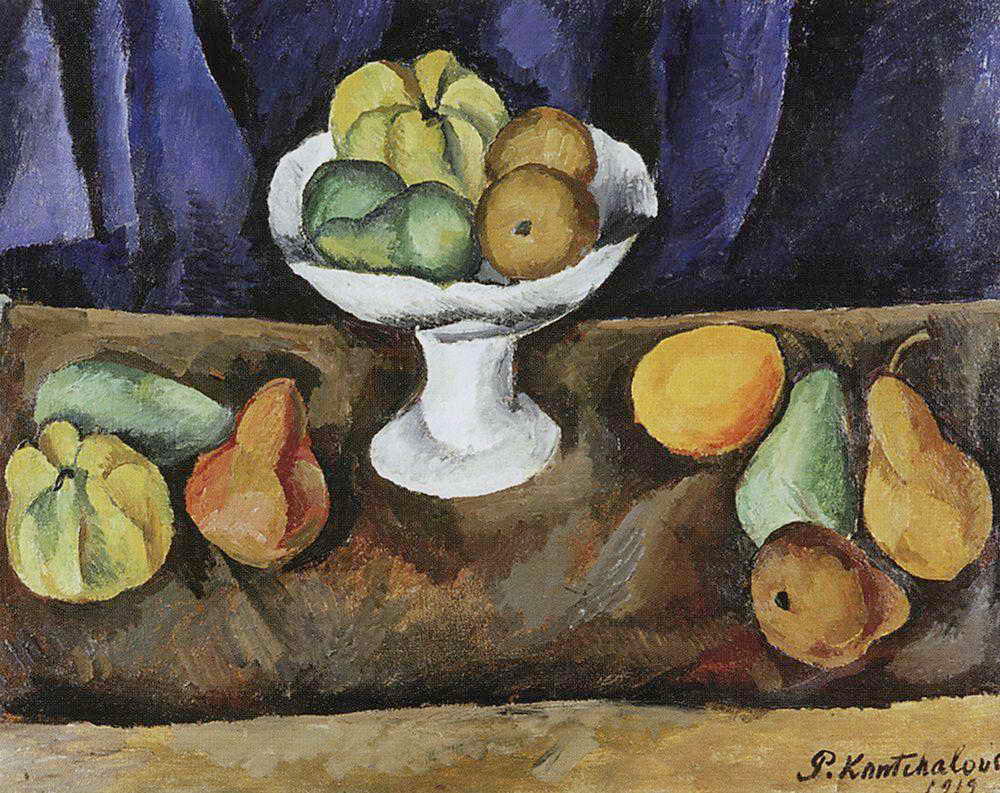The image is a detailed still life painting of fruit, created in 1919 by an artist whose name is difficult to read but might be something like G. Knntchaloue. The medium of the painting is uncertain but it appears to be either watercolor or oil based on the texture and finish. The central focus of the artwork is a white pedestal bowl that sits on a crudely drawn brown table. The bowl contains various misshapen fruits, including pears, oranges, and possibly a mango or small gourd. These fruits are vividly colored in greens, yellows, oranges, and reds. Additional fruits and vegetables are scattered on the table to the left and right of the bowl. The background features a coarse, dark blue curtain or tapestry, which adds a contrasting backdrop to the vibrant colors of the fruit and the stark white of the bowl. This painting, characteristic of a still life composition often seen in beginner art classes, emphasizes form, color, and arrangement in a simplistic yet captivating manner.